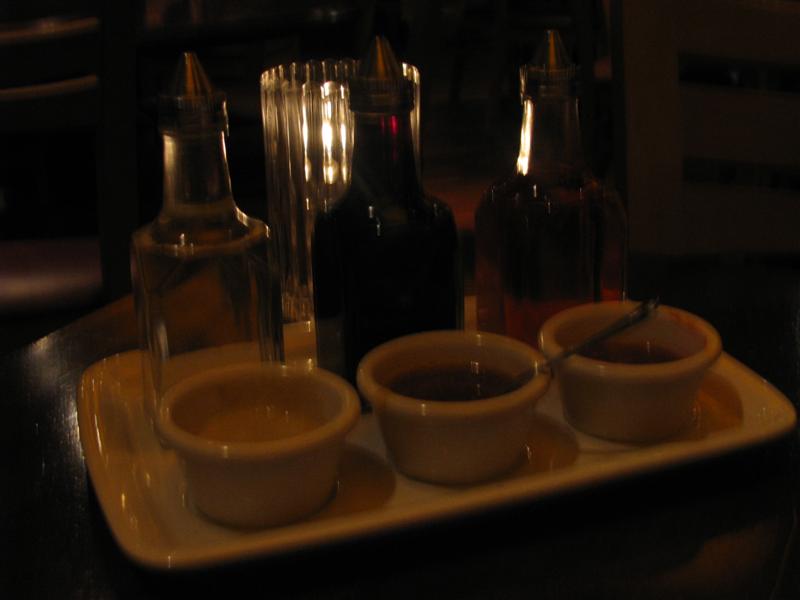This photograph depicts a calming setting with a dark yet warmly-lit ambiance, reminiscent of a spa or an herbal tasting room. The focal point is a glossy, yellow-painted concrete tray placed on a black table. On this ceramic tray are three transparent glass bottles, each with a conical metal dispenser cap.

In front of each bottle, positioned horizontally along the tray, are three ramekins. The ramekin on the left contains a yellow sauce. The middle ramekin, which has a silver spoon resting in it, holds a brown sauce. The third ramekin, to the right, contains a reddish-brown sauce with some reddish stains on its sides. Each ramekin appears to be associated with the liquid in the bottle behind it.

At the back of this arrangement, a glass is positioned to catch and reflect the room's orange lighting, further enhancing the tranquil atmosphere. The setting suggests an experience dedicated to tasting or sampling, possibly featuring oils or natural remedies.